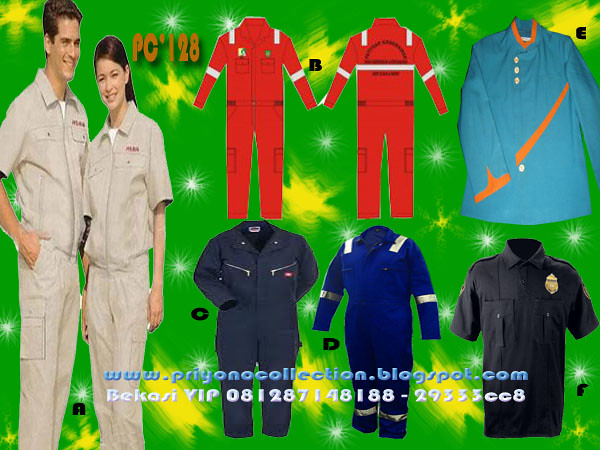This image appears to be an advertisement for various uniforms. The backdrop is green with abstract yellow star-like bursts and white letters reading "PC128." On the left side, there is a man and a woman, both with brown hair and dressed in light beige one-piece janitor uniforms. The man stands on the far left with a tilt and his right hand in his pocket, while the woman smiles beside him. Below them is a website link, pryonoccollection.blogspot.com, and additional labeling indicating this is likely not an American company.

On the right side of the image, there are two rows of three uniforms displayed. The top row includes a red and white uniform in the center, showcasing both the front and back, flanked by a blue tunic with an orange collar and stripe on the right. The bottom row features a navy blue jumpsuit on the left, a light blue jumpsuit with white shoulders in the center, and a black shirt with a golden badge on the chest on the far right. This suggests the ad is promoting a wide range of uniforms, likely for professions such as security, fire service, or culinary work.